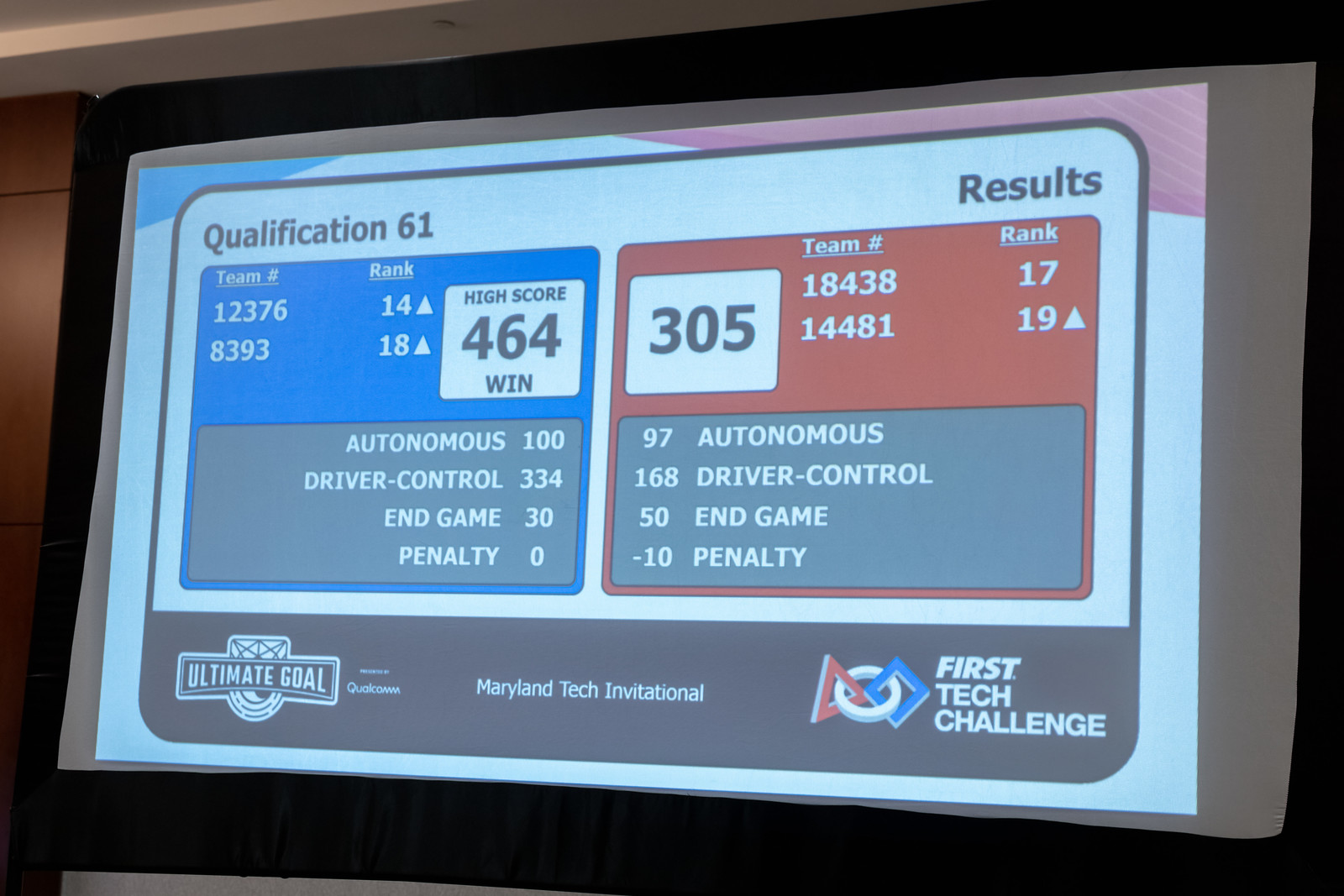The image captures a screen from the First Tech Challenge at the Maryland Tech Invitational. In the lower right corner, the First Tech Challenge logo—composed of three interconnected shapes in red, white, and blue—is prominently displayed. To its left, “Maryland Tech Invitational” and “Ultimate Goal Qualcomm” are clearly labeled.

In the upper left section of the screen, the text "Qualification 61" is displayed in black letters within a white rectangle bordered in black. Below, a blue box lists team numbers and their ranks: Team 12376 is ranked 14, and Team 8393 is ranked 18. An adjacent white box highlights their high score of 464, indicating a "win." Performance details further include Autonomous: 100, Driver Control: 334, End Game: 30, and Penalties: 0.

To the right, a red box marked "Results" displays further team statistics. Team number 18438 is ranked 17, and Team 14481 is ranked 19, each with an upward arrow. A white rectangle featuring the number 305 is placed alongside these team details. Below in a gray box, additional scores are listed for this team: 97 for Autonomous, 186 for Driver Control, 50 for End Game, and -10 for Penalties.

Overall, the screen conveys detailed performance metrics and rankings of teams in the competition, providing a comprehensive view of the standings and scores in the First Tech Challenge.